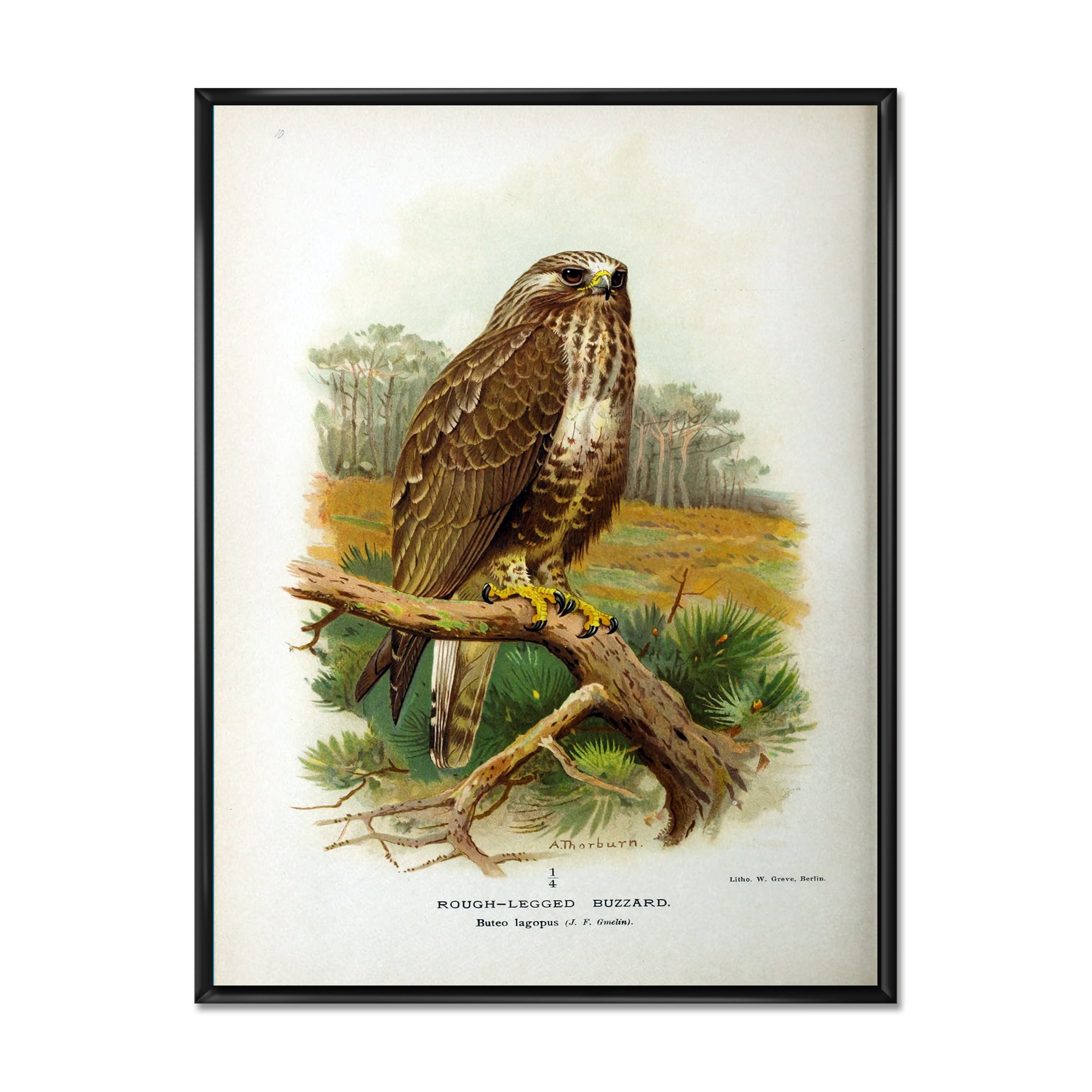This detailed framed illustration presents a Rough-legged Buzzard (Buteo lagopus), often mistaken for an owl, meticulously drawn by the artist A. Thorburn and published by Lithow W. Grove Berlin. The buzzard is perched gracefully on a prominent tree branch, showcasing its intricate brown feathers with white stripes, brown eyes, and a yellow area surrounding its sharp black beak. The majestic bird balances with its yellow taloned feet grasping the branch. The background depicts a natural landscape with trees, patches of yellow and green foliage, and an overall dry environment, contrasting against a white sky. The entire artwork is encased in a black frame, adding to its elegant presentation.